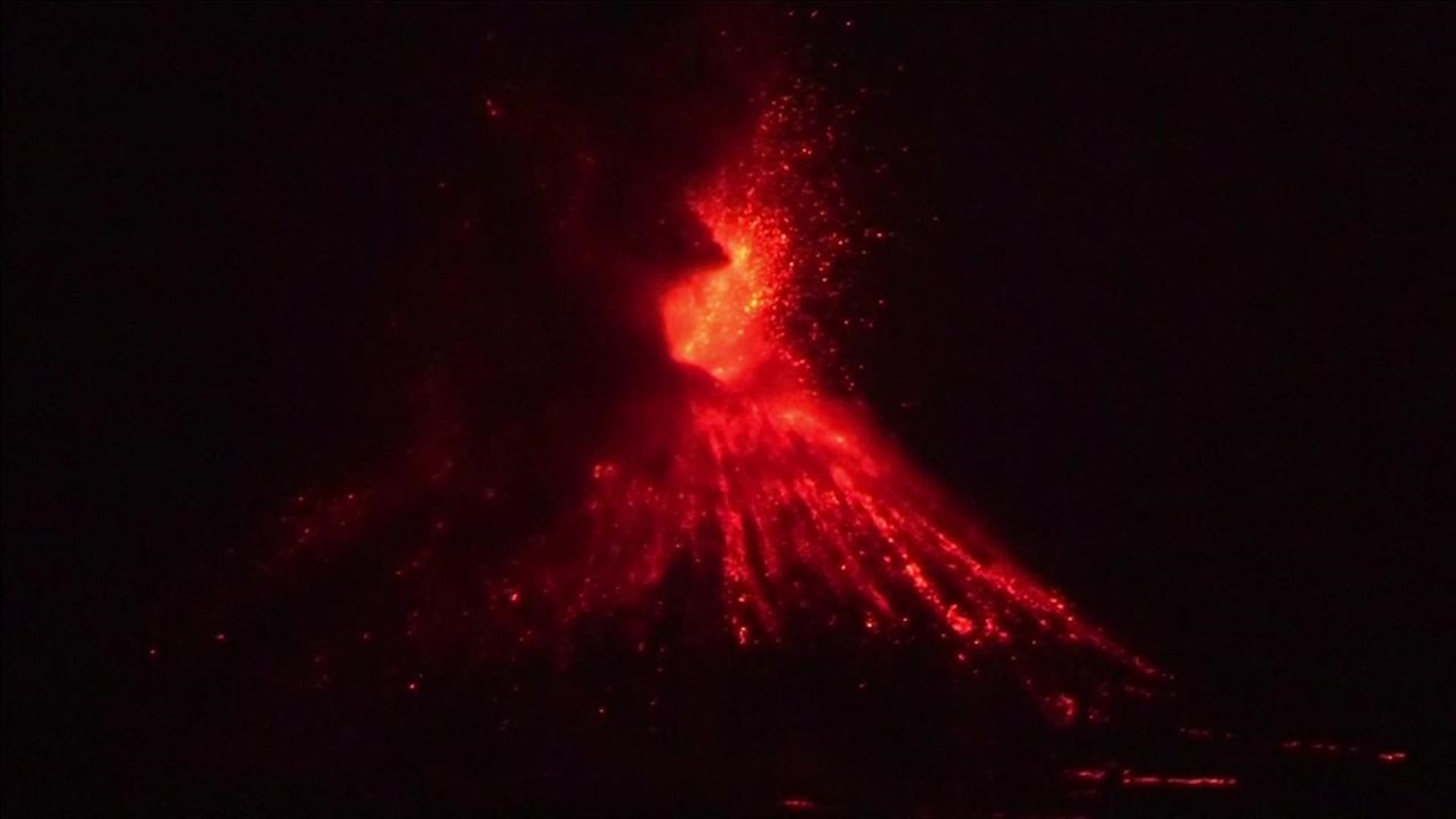Captured at night, this horizontal photograph reveals a volcano in full eruption. The predominantly dark image is punctuated by the bright, fiery red and orange lava spewing from the volcano's top. Particles of bright lava erupt upwards into the sky and trail down the mountain's sides. Thick, black smoke obscures part of the scene, especially to the left of the volcano. Some lava flows down to the base of the volcano, visible at the bottom right of the image, creating a glowing path amidst the surrounding darkness.